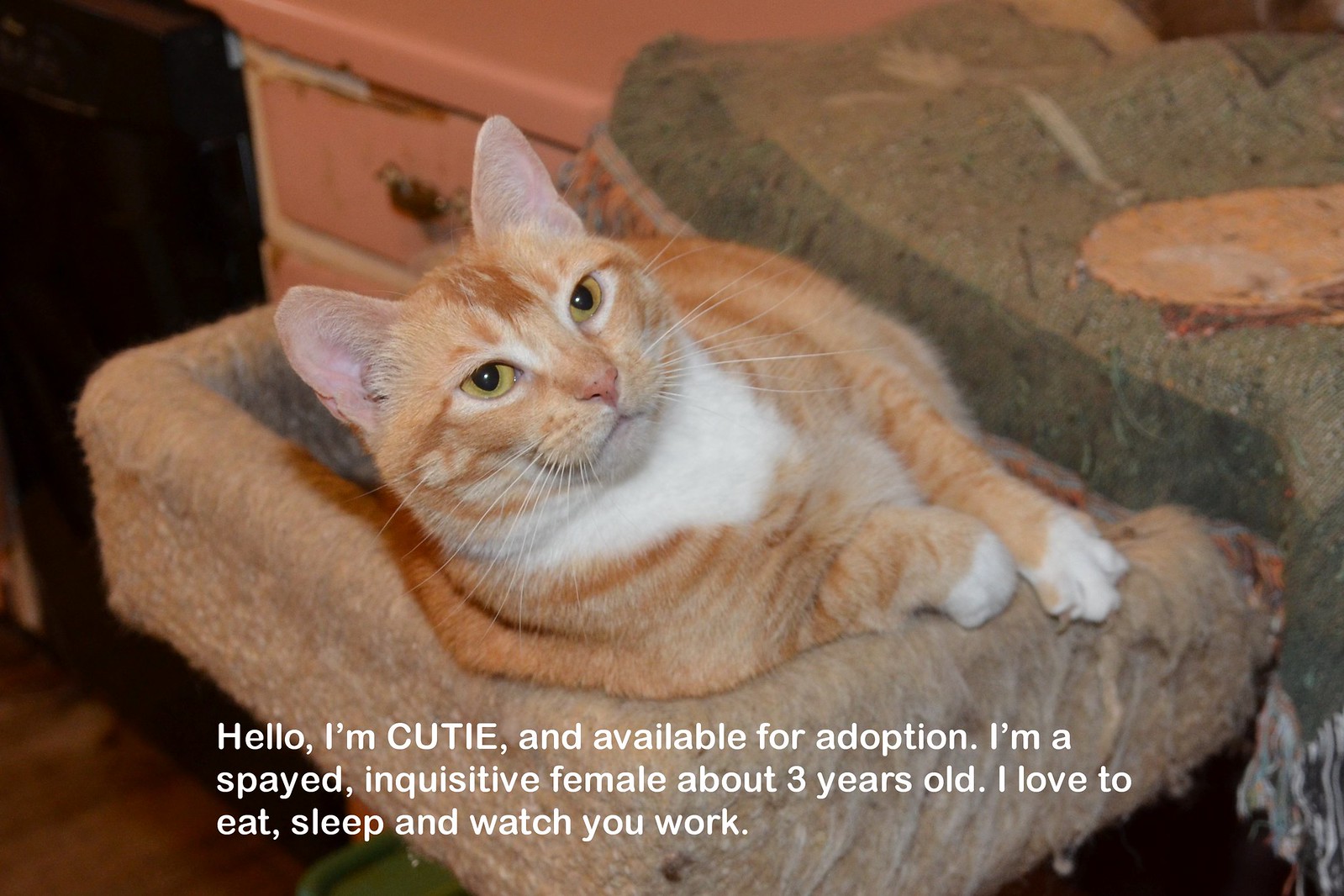In this detailed photograph taken indoors, a brown and white tabby cat is the focal point, sitting comfortably in a light brown, square cat bed right in the center of the image. This inquisitive feline, with striking black and yellow eyes, a pink nose, pink ears, and white paws, gazes off into the distance. The cat bed appears to be made of a soft material positioned on what seems to be either a wooden or hard surface floor. Directly behind the cat, there's a pink-colored table, and to the right, a gray blanket or cloth is visible. The background also includes a dresser and another bed, adding to the cozy setting. White text at the bottom of the image reads, "Hello, I'm Cutie and available for adoption. I'm a spayed inquisitive female, about three years old. I love to eat, sleep, and watch you work." This image appears to be part of an advertisement for an adoption agency, showcasing this adorable cat's serene and endearing nature.